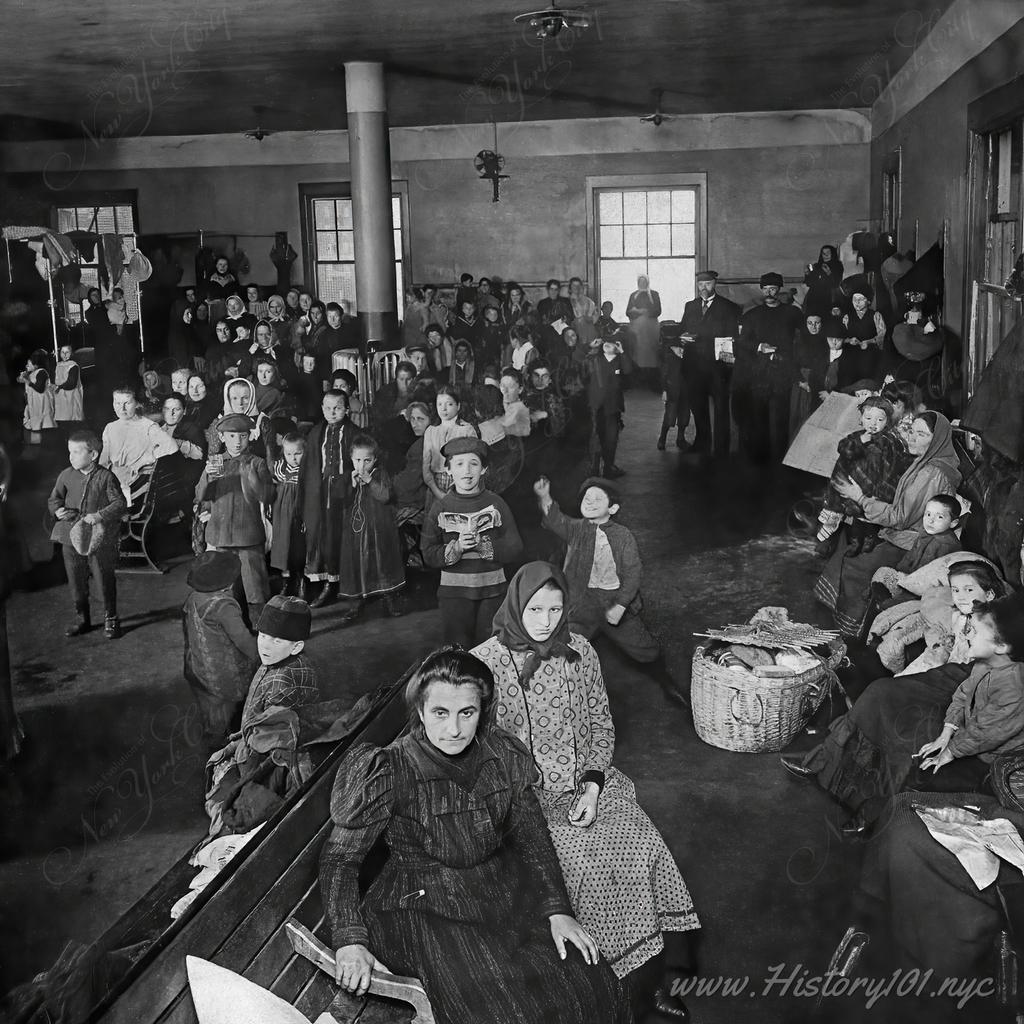This black and white photograph, likely from the early 1900s, captures a poignant scene of a large group of people gathered in what appears to be a waiting area, possibly at Ellis Island or a similar transit location for immigrants. The image, shaped as a slightly taller-than-wide rectangle, exudes a historic ambiance amplified by its grayscale tones. The room is spacious yet sparsely furnished, with a prominent metal pole or column on the left side and several wooden benches. 

Among the crowd are numerous children, dressed in period-appropriate attire—girls in long dresses, boys in suits and hats. Many women are seen wearing headscarves, suggesting Eastern European origins. The people are seen either sitting on benches, standing around, or leaning against the walls. The background reveals a few windows and potential indicators of the building’s age, such as oil lamps hanging from the ceiling and possibly an early electric fan on the wall.

The photograph's evocative detail, ranging from the clothing styles to the somber expressions, paints a vivid picture of an immigrant experience. At the bottom of the image, the watermark “www.history101.nyc” indicates its archival source.